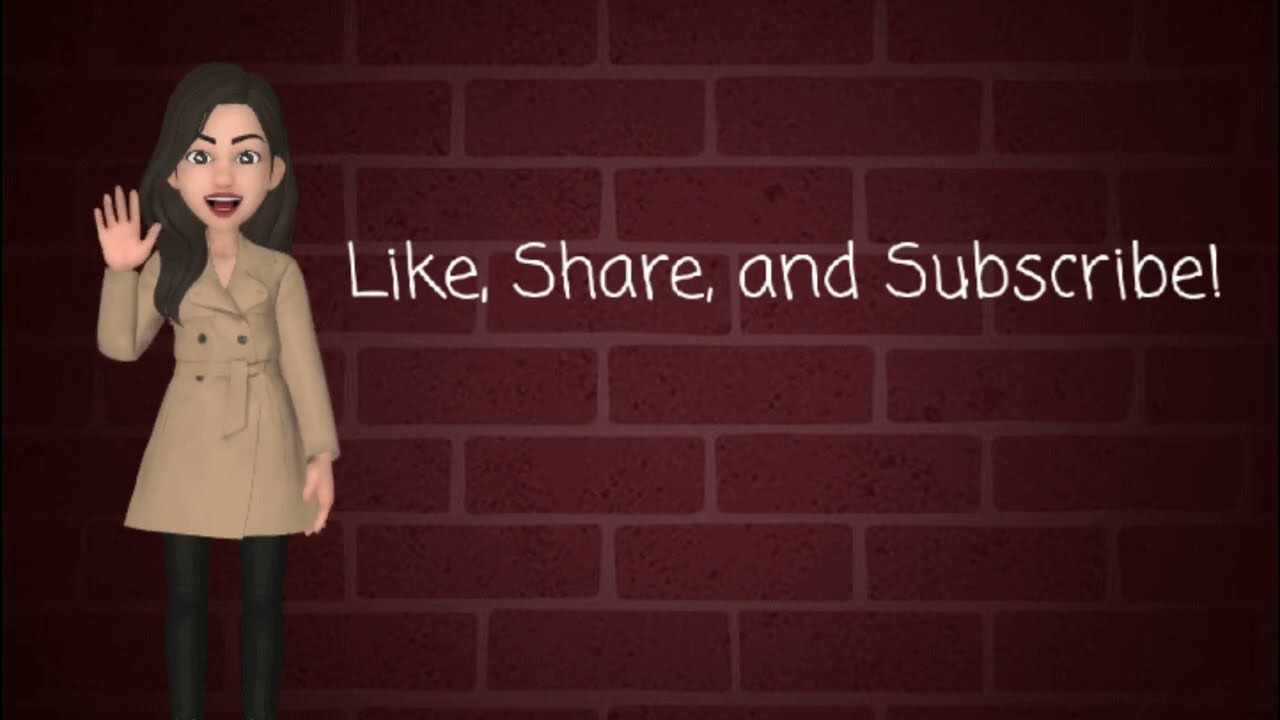Set against a dark red brick wall, this image features an animated drawing of a woman with long brown hair, brown eyebrows, and brown eyes. She's smiling with her mouth open, giving a friendly wave with her right hand raised, palm facing forward. Dressed in a cream-colored trench coat with a tied belt, black leggings or pants, and red lipstick, she appears to be casually inviting viewers in. The woman's left arm is held straight down by her side. To her right, in the center of the image, the words "Like, Share, and Subscribe!" are prominently displayed in handwritten-style white text, likely intended to encourage audience engagement. The atmosphere of the image is somewhat dim due to the darker tones, yet the white text and the woman's vibrant features stand out vividly against the backdrop.